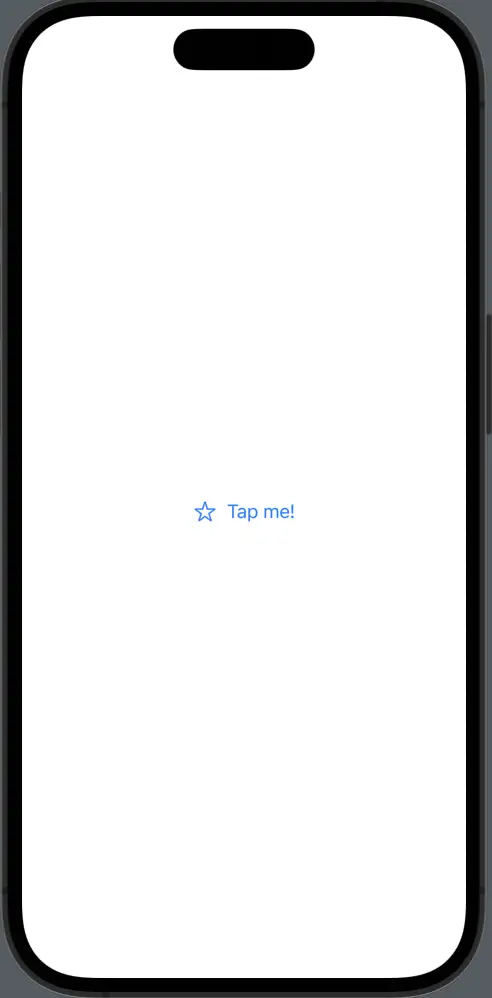The image depicts a screenshot of a phone, captured in a portrait orientation. The phone is set against a gray background, though only slivers of this backdrop are visible along the thin corners on the right side, as the captured image is quite large. The phone itself is a black, rectangular device with rounded edges. 

On the phone's screen, which is predominantly white, there is a noticeable dark oval at the top, likely designed to house the camera or other sensors. In the center of the screen, there is a blue star outline with a transparent white interior. Directly below the star, the text "Tap me!" is displayed in blue. 

The rest of the screen remains blank and white, giving the impression that either the application or display captured is incomplete or experiencing a glitch. The purpose of the lone star and text is unclear, as there are no additional buttons, links, or instructions. This sparse screen suggests that tapping on the star might trigger an action or reveal additional content, though what that might be isn't evident from the image alone.